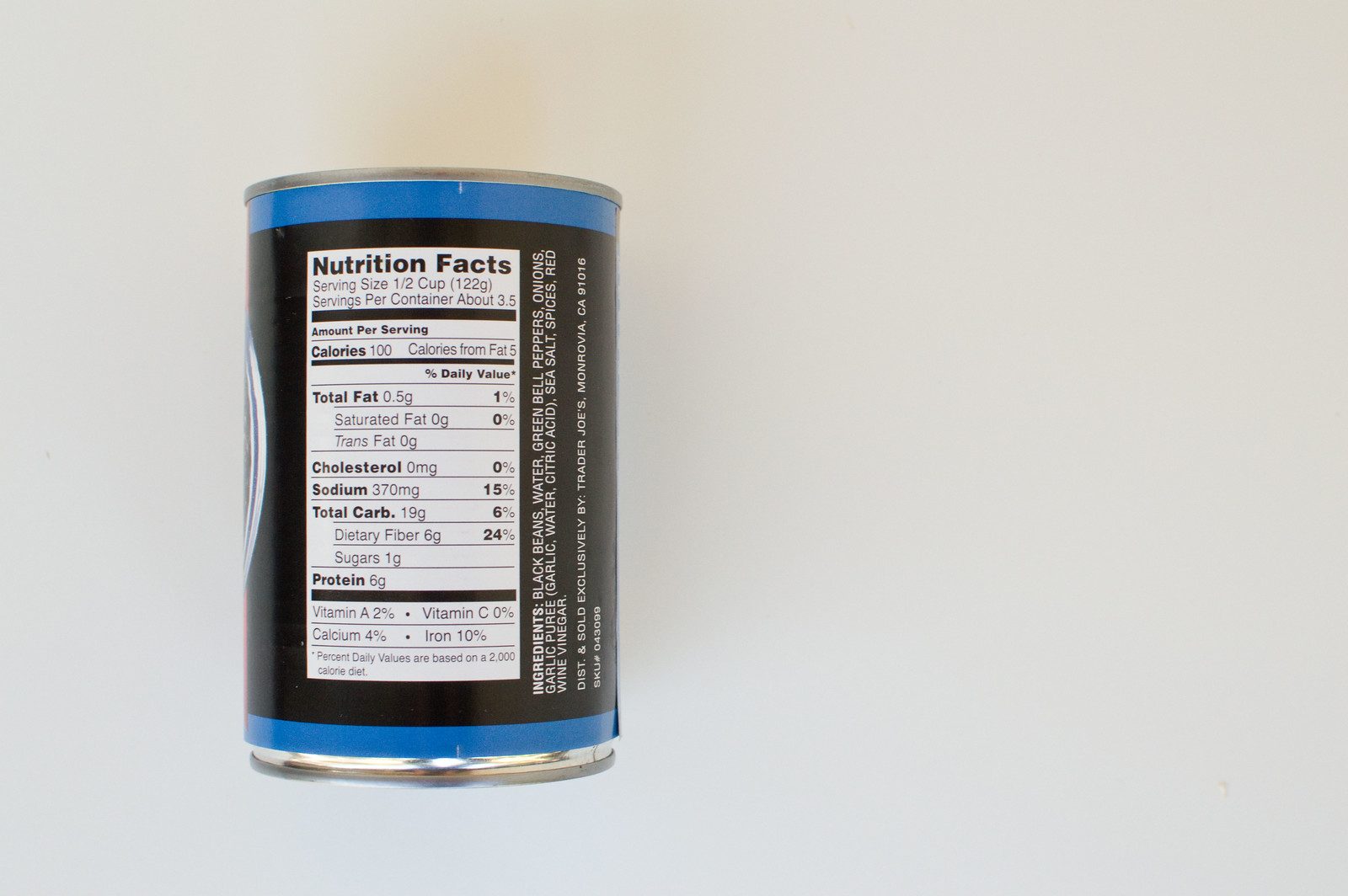This image features the back of a black and blue aluminum can of Trader Joe's black beans, positioned against a light gray background. The can has a blue ring at the top and bottom and features a large white box labeled "Nutrition Facts" in black writing. The nutritional information indicates a serving size of half a cup (122 grams), with about 3.5 servings per container and 120 calories per serving. Detailed nutritional values include 0.5 grams total fat, 0 grams saturated fat, 0 grams trans fat, 0 milligrams cholesterol, 15 milligrams sodium, 24 grams total carbohydrates, 6 grams dietary fiber, 1 gram sugars, and 6 grams protein. Additionally, it lists 2% Vitamin A, 4% Calcium, 10% Iron, and 0% Vitamin C. The ingredients, written sideways, include black beans, water, green bell peppers, onions, garlic puree, garlic water, citric acid, sea salt, spices, and red vinegar.